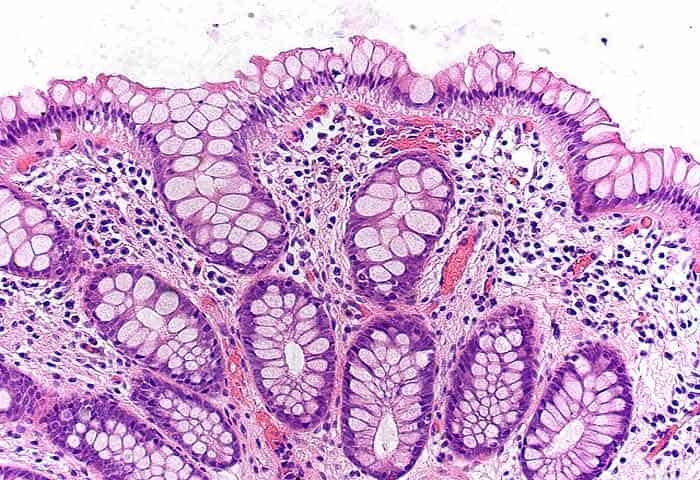This image presents an artistically rendered or computer-imaged microscopic view of an organic material, possibly a tissue sample stained in reddish-purple hues. The medium-quality image, measuring approximately 8 inches by 6 inches, lacks a border or text. It features a complex structure of cellular-shaped nodules and tiny connectors, interspersed with dark blue granule blobs. The round cell walls and varying cell types suggest it is not plant tissue, but rather a biological specimen, potentially animal tissue or blood cells. The visual complexity and color staining make it resemble images seen in scientific textbooks, possibly related to cancer diagnostics or cellular studies, though the exact nature of the sample remains unclear.